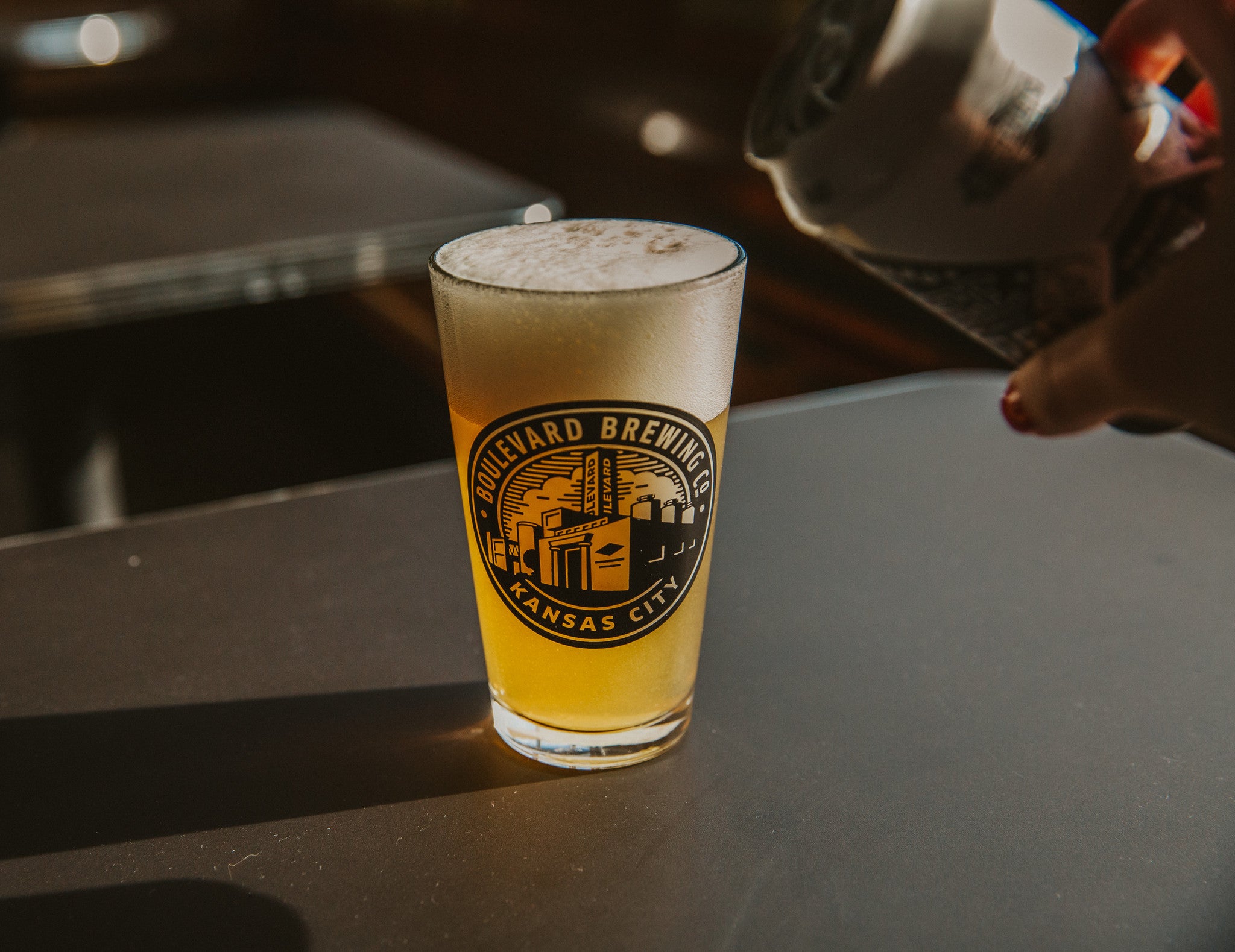A photograph captures a pint glass of beer prominently placed on a dark gray table, suggesting a bar-like setting. The pint glass, bearing a lush, foamy head and filled with a light yet slightly hazy amber beer, features a circular logo in a 50s industrial style. This logo, which reads "Boulevard Brewing Company, Kansas City," depicts a small industrial building, presumably the brewery itself. The scene appears to be set in an evening, inferred from the dim lighting and the shadows cast by the glass. A woman's hand with red nail polish, slightly out of focus, is seen pouring beer from an aluminum can that shares the same logo as the glass, adding a dynamic element to the otherwise still composition.